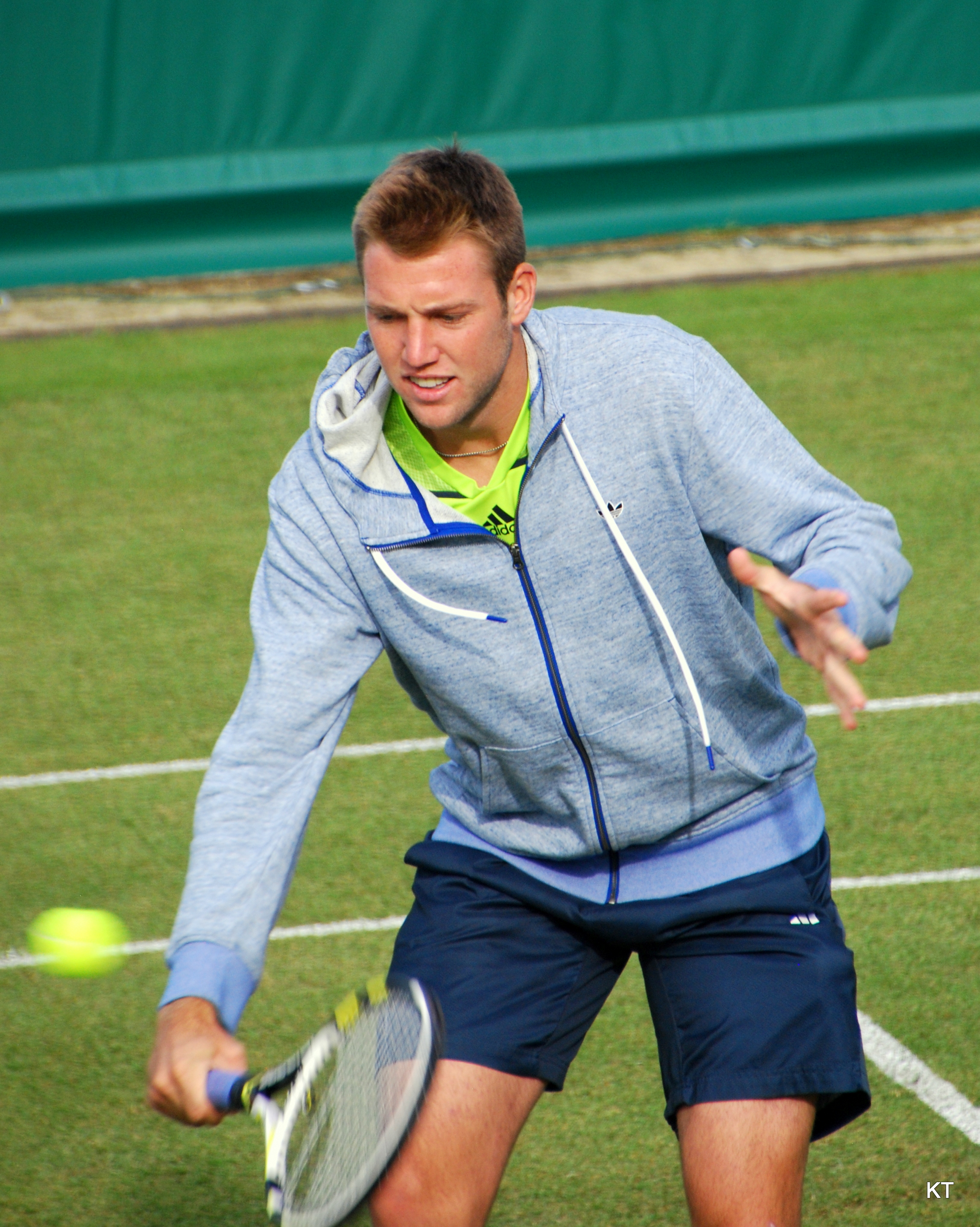This image showcases a tennis player in action, positioned at the center of the frame. He is wearing a light gray-blue, mottled zip-up hoodie with a blue zipper, and beneath it, a neon-green shirt adorned with a black Adidas logo. His dark blue shorts add to his athletic attire. The player has short brown hair and is intently focused on a blurry, green-yellow tennis ball that hovers slightly above and to the left of his white tennis racket, suggesting that he has either just hit the ball or is about to strike it. His left hand is outstretched with open palms while his right hand firmly grips the racket in a low position. He stands on a grassy astroturf tennis court with thin, white lines delineating the playing area. In the bottom right corner of the photo, the initials "K.T." can be seen in white letters. The background includes a cyan-blue-green wall, completing the setting of this dynamic sports moment.